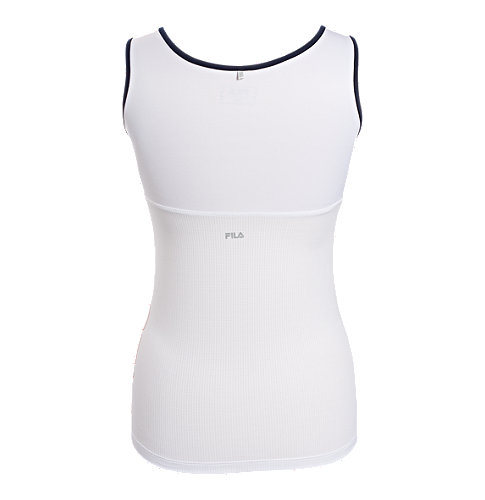This product image showcases a women's athletic tank top, likely intended for high-movement activities such as running. The top is predominantly white with a body-hugging, form-fitting design that accentuates an hourglass shape by curving inward at the waist and flaring slightly at the hips and shoulders. The neckline and armholes are trimmed with black or navy blue, providing a striking contrast to the white fabric. A horizontal seam runs beneath the bust line, suggesting the possibility of an integrated sports bra. The top features the brand name "Fila" in small silver text prominently positioned near the navel area. Additionally, there is a subtle symbol around the midsection, akin to where a necklace would rest. Positioned against a completely white background, this image is likely the primary product shot used for online retail platforms such as Amazon, effectively highlighting the garment's design and branding.